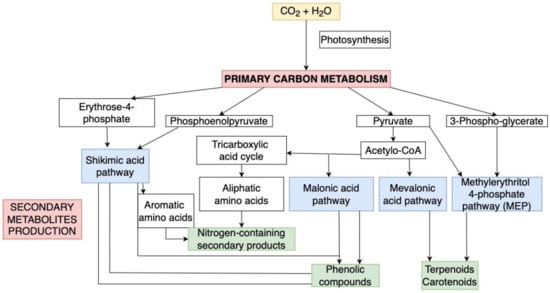The image is a detailed flowchart set against a pure white background, depicting the various stages of photosynthetic and metabolic pathways. At the top, a yellowish block labeled "CO2 + H2O" leads down via a black arrow to a white block that says "photosynthesis." This white block connects further down to a light reddish block with thick black text that reads "primary carbon metabolism." From this point, four arrows branch out in various directions:

1. **Left Pathway:** The first arrow leads to a white block named "erythrose-4-phosphate," which then points to a light blue block labeled "shikimic acid pathway." Two arrows from this pathway diverge, one going to a green block titled "phenolic compounds" and another to a white block saying "aromatic amino acids," which continues to a green block named "nitrogen-containing secondary products."

2. **Second Pathway:** Another arrow from the primary carbon metabolism block leads to a white block labeled "phosphoenolpyruvate," which follows again to the "shikimic acid pathway." 

3. **Third Pathway:** A downward right arrow points to "pyruvate," leading to two subsequent branches. One path goes right to a blue block saying "methyl erythritol for phosphate pathway (MEP)," leading further to another green block labeled "terpenoids and carotenoids." The other path heads downward to "acetyl-CoA," which points to another blue block titled "mevalonic acid pathway," also leading to the green "terpenoids and carotenoids" block.

4. **Fourth Pathway:** The far-right arrow points to "3-phosphoglycerate," leading to the "MEP pathway" and subsequently to the green "terpenoids and carotenoids" block.

Additionally, the "acetyl-CoA" box also links through a blue block labeled "mevalonate pathway" to the "phenolic compounds" green box. The entire diagram is sprinkled with light blue blocks indicating various pathways and light reddish blocks guiding primary and some secondary processes, concluding with a focus on "secondary metabolites production" on the lower left.

Overall, the diagram meticulously illustrates the complex interactions and transitions in photosynthetic and metabolic processes, displayed through color-coded blocks and arrows.